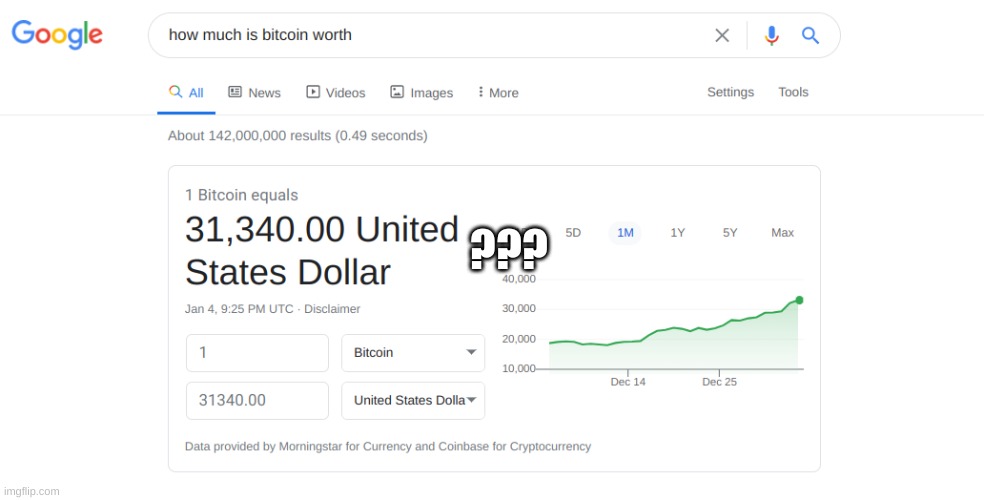An edited screenshot of a Google search result. Prominently featured at the top left is the Google logo, followed by a search bar to its right, containing the query “how much is Bitcoin worth” in lowercase letters. Below the search bar, the main search result indicates that 1 Bitcoin equals $31,340 USD, with question marks superimposed over this part of the image. Adjacent to the dollar amount, a small green line graph depicts Bitcoin's value trajectory over time. In the bottom left corner, underneath the stated Bitcoin value, there is a small text box displaying the number one. To its right, a drop-down box is set to Bitcoin. Beneath this, another text box displays the dollar amount, paired with a drop-down box indicating United States Dollar. At the screenshot's bottom right corner, small gray text credits "data provided by Morningstar for currency and Coinbase for cryptocurrency." Additionally, in very tiny letters at the extreme bottom right, the URL "mflip.com" is visible.